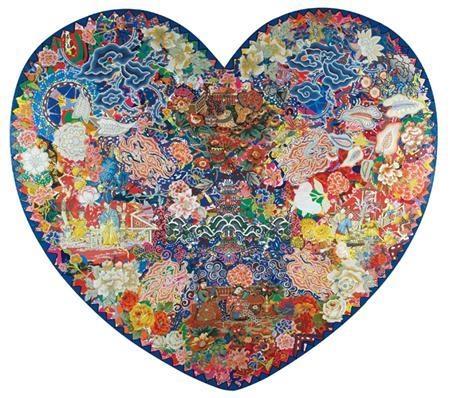This heart-shaped image, bordered in a dark blue, is a small, dynamic mosaic filled with vibrant colors and intricate floral patterns. While there is no outer border, the heart itself is set against a dark blue background. The design features an abstract assemblage of flowers and shapes in a rich palette of blues, greens, reds, yellows, whites, pinks, and oranges. The top of the heart is dominated by blue hues, with white and red accents interspersed throughout. Notably, red details appear at both the top and bottom points of the heart. The flowers and patterns, including roses and various unnamed blooms, create a quilt-like effect with swirling, wavy, and curvy lines. The edges of the heart are made up of small, pointed triangles contributing to its textured appearance. Some areas of the pattern hint at faces or human-like figures dressed in Asian-inspired gowns, adding a layer of mystique and cultural impression to the image. The intricate swirl and wave patterns within the heart give it a lively and engaging look, with colors blending harmoniously and standing out vividly.